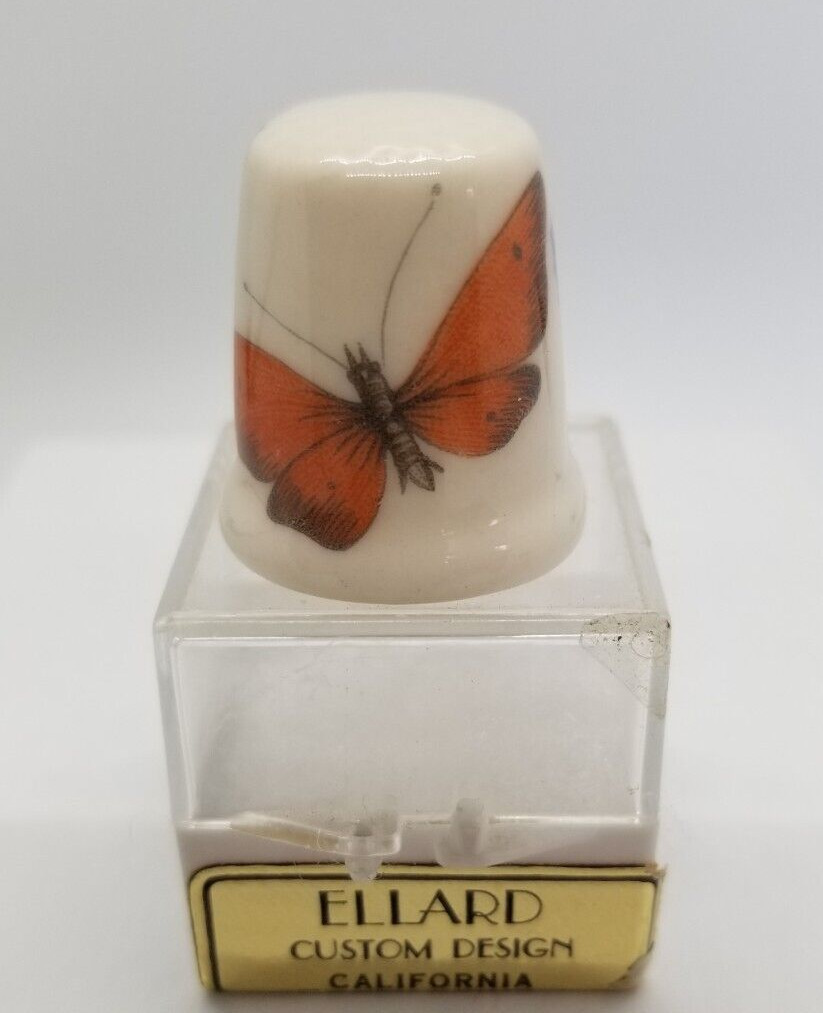This image depicts a candle placed on top of its container. The container has a cube-shaped, translucent body, resembling glass or clear plastic. At the bottom of the container, there is a gold label with black trim displaying the inscription "Eliad Custom Design, California." The candle itself is white and features a prominently large butterfly design on its surface. The butterfly has brick-red wings with black edges and a black body. Additionally, there appears to be a cup turned upside down on the container, further enhancing the intricate presentation. The background of the image is off-white and gray.